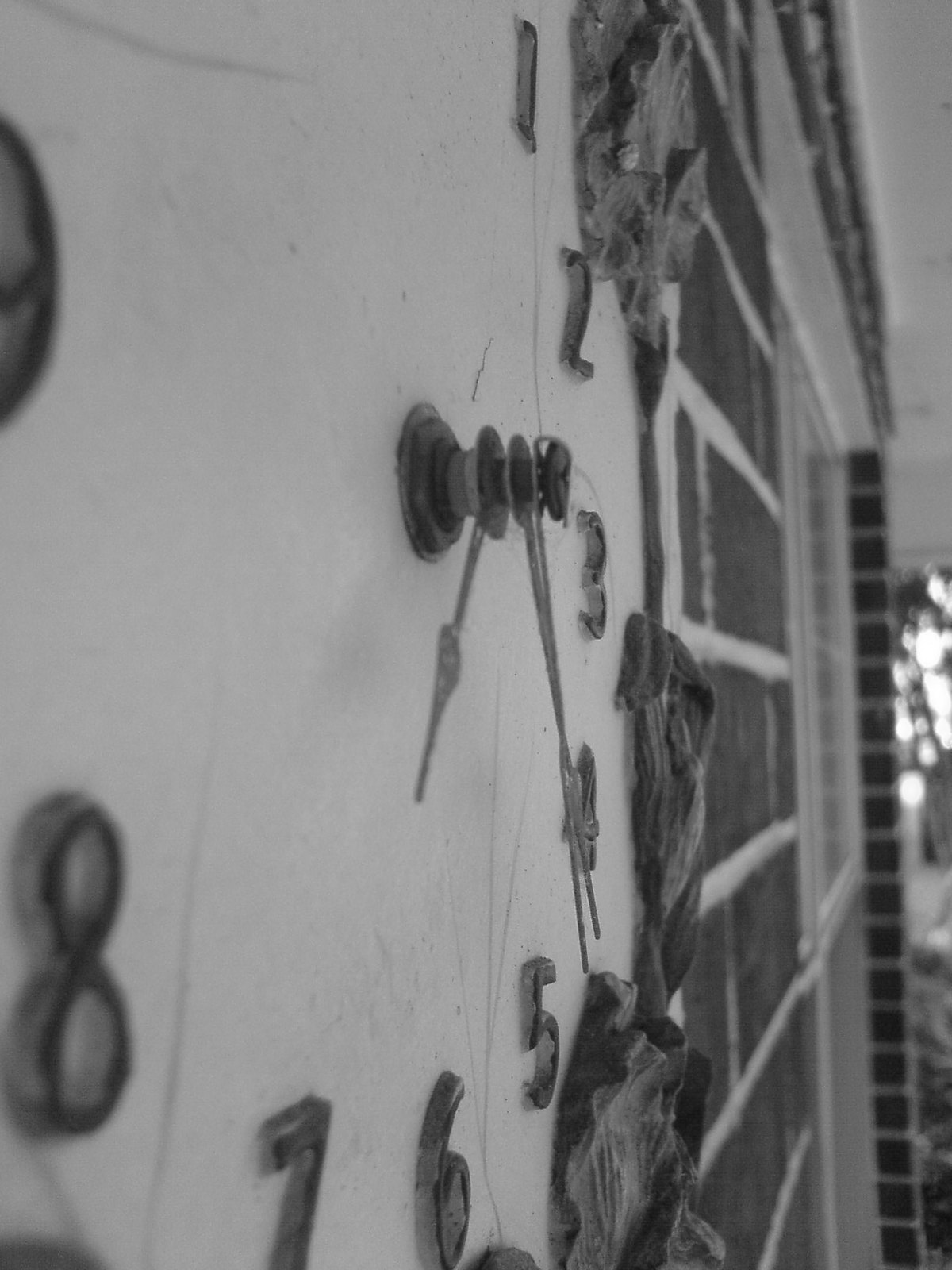This black-and-white photograph captures an intriguing side view of a wall clock, zoomed in closely to the central bolt where the clock's hands are attached. The clock face is white, featuring bold, black numerals that stand out crisply against the light background. The image is taken from a unique angle, almost as if the camera were pressed against the face of the clock, slightly askew. Enhancing the clock's aged ambiance, it hangs on a brick wall, which appears to be partially covered in foliage or perhaps cobwebs. The blurred, textured surface in the background suggests the clock might be affixed to the exterior side of a brick house.